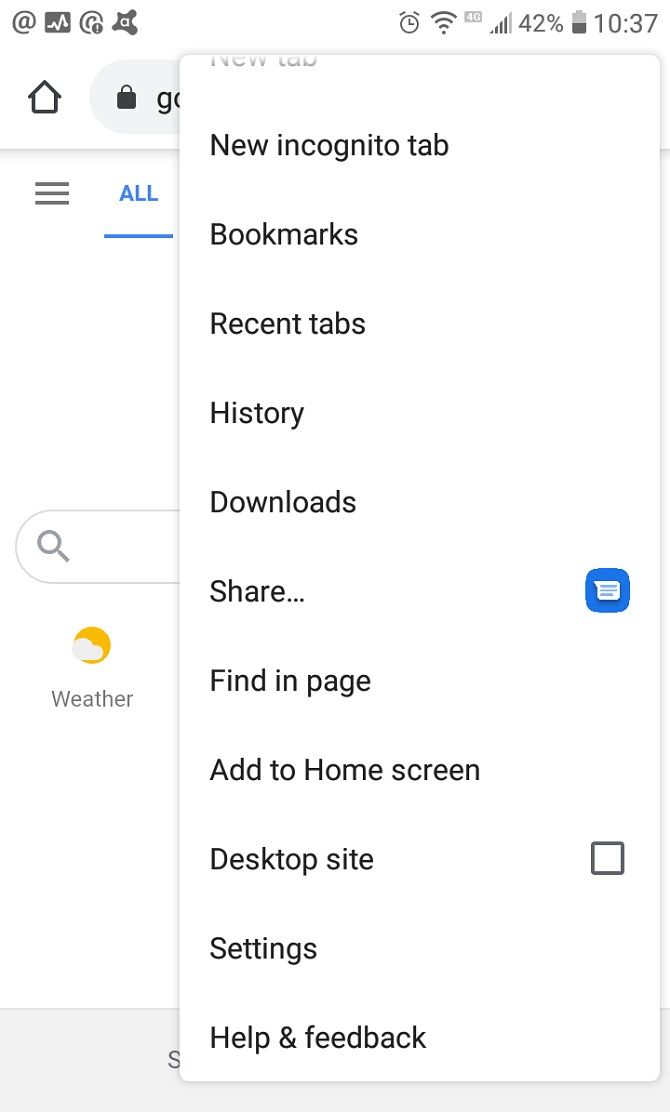A detailed screenshot of a mobile device, possibly a smartphone or tablet, depicting the current state of its screen. At the very top, various status icons are visible, including an alarm icon, a Wi-Fi symbol, a 4G network indicator, a battery icon displaying 42% charge, and the current time, 10:37. 

The main backdrop features a web browser, evidently Google Chrome, as suggested by the partially visible URL starting with "geo." While the majority of the browser's URL bar is obstructed by an overlaid menu box, we can infer the web page being accessed.

The overlay is a white pop-up menu with black text, opened up from clicking the three vertical dots (ellipsis) typically located at the top-right corner beside the profile avatar. The menu includes the following options: "New incognito tab", "Bookmarks", "Recent tabs", "History", "Downloads", "Share" marked by an ellipsis and a downwards pointing speech bubble icon in blue, separated by a blue highlighted edge, "Find in page", "Add to home screen", "Desktop site" indicated by an unchecked square box, "Settings", and "Help & feedback".

Also visible in the background is a weather icon, providing quick access to the local 5-day weather forecast via Google. The screenshot captures an active, engaged browsing session likely taking place on a Google search or web page.